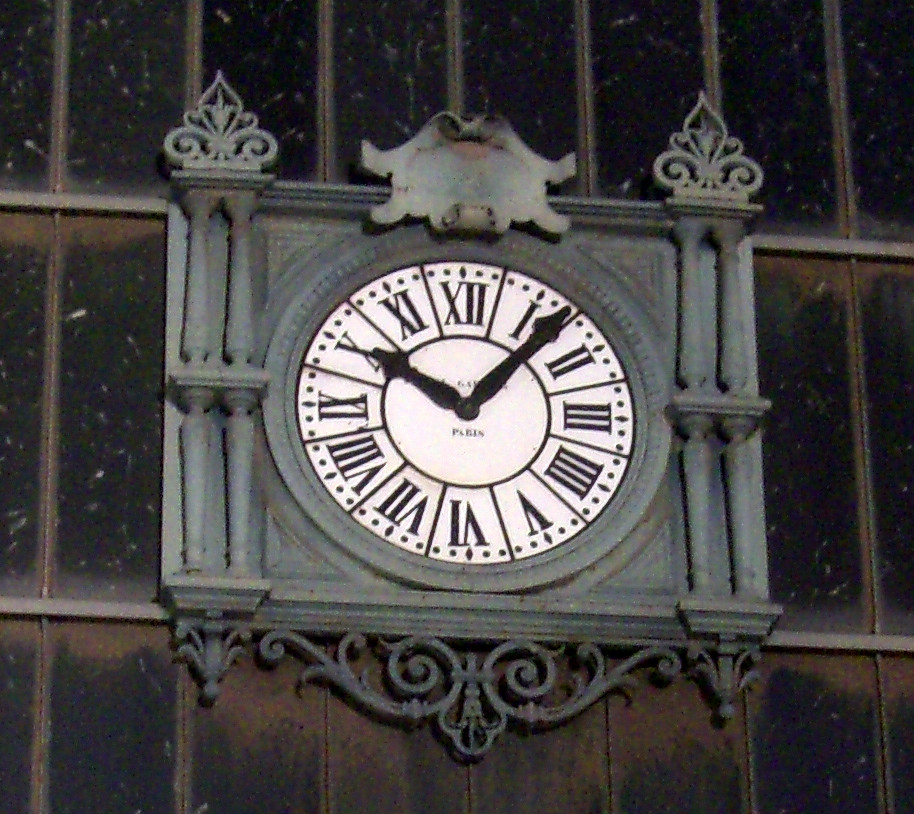This photograph captures a close-up of a large, ornate clock mounted on the side of a dark, Gothic-style building. The clock, which appears to be slightly aged, is encased in a grand square gray frame adorned with intricate details. Four ornate columns frame the sides, while delicate iron railings and fleur-de-lis-inspired patterns embellish the upper section. The clock face itself is a pristine white, featuring prominent Roman numerals and minute dots that encircle the perimeter. The hands of the clock point to approximately 10:09. The dark hue of the building's facade contrasts sharply with the clock's lighter elements, further highlighting its elaborate design.